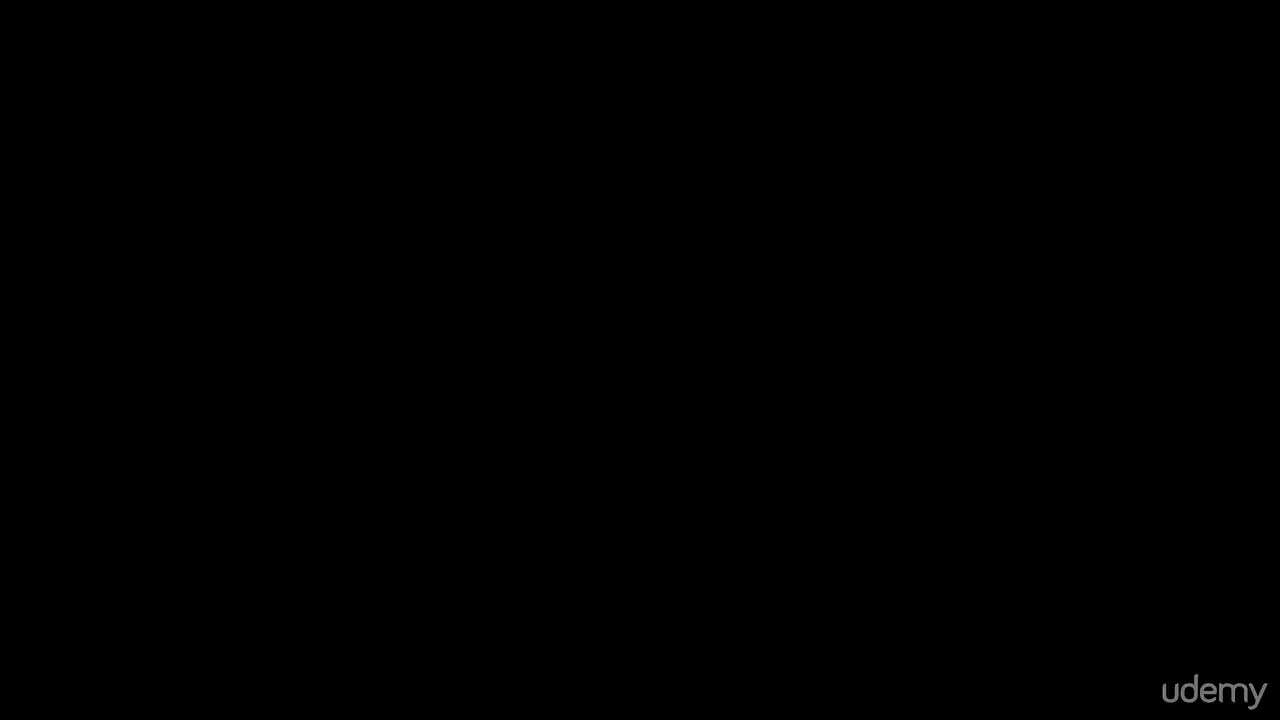The image is a screen capture of an older computer screen displaying two overlapping windows. The top window features a blue banner with white text that reads "Select Process to Attach." This dialog box includes a table with columns labeled PID, Name, Service, Listening, Window, and Path, filled with various entries, where PID numbers are in white text. The table itself displays green text on a black background, reminiscent of an MS-DOS interface. Below this window, part of a larger application screen is visible, containing menu items such as Plugins, Immlib, Options, Window, Help, and Jobs along the top, with "Immunity: Consulting Services Manage" noted on the upper right. In the lower left corner of the entire image, the word "UDEMY" appears in off-white, slightly superimposed text. The overall aesthetics of the computer screen and the interfaces give it a vintage, rudimentary Windows appearance.